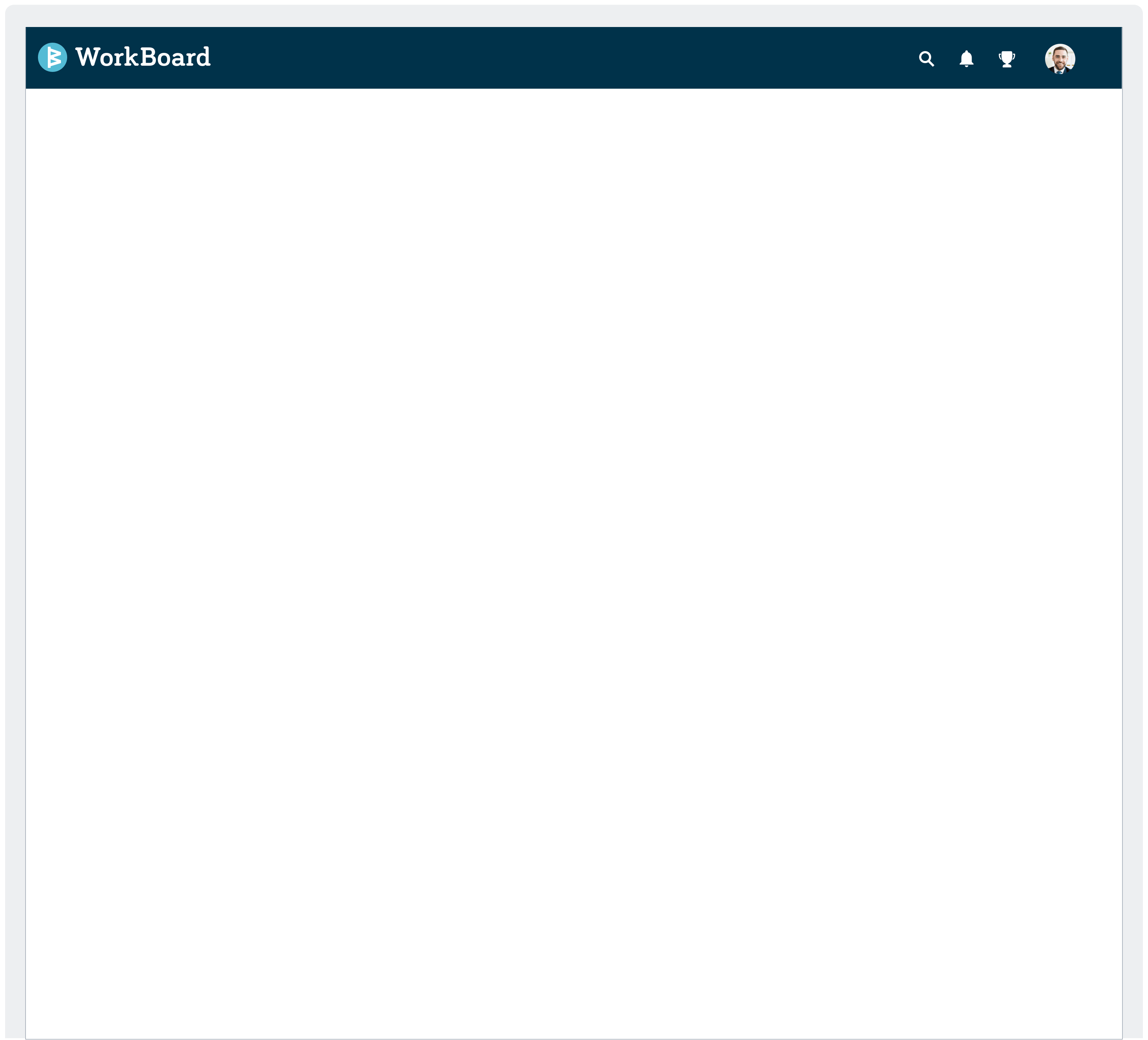A screenshot depicts a blank page with a minimal number of items positioned at the top left corner. The header is adorned with a greenish-blue and black banner, featuring an icon resembling two small flags followed by the text "Work Board." On the extreme right side of the header, there are several icons: a search icon, a bell icon, a trophy icon, and lastly, a circular icon with a front camera-style photo of a man in a suit against a beige background.